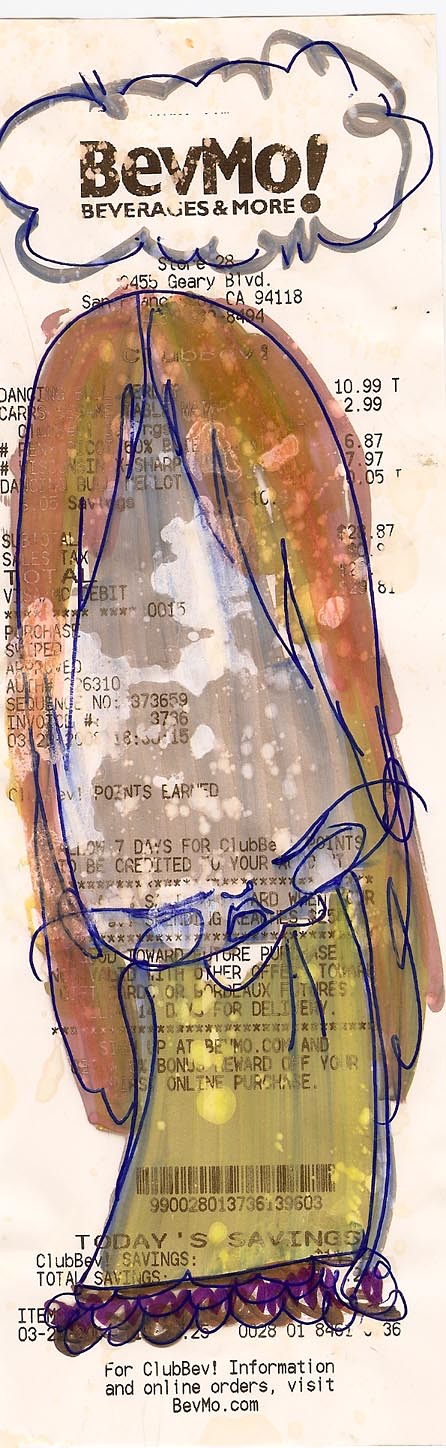A cropped image of a BevMo receipt, partially covered by a large drawing that appears to be either an oil painting or a watercolor. The edge of the receipt rests on a white surface, possibly a tabletop. The top of the receipt features "BEVMO!" in bold, brown letters, with "Beverages and More" centrally aligned beneath it. The store name is circled with a blue pen, which has been outlined with a gray color. Despite most of the receipt being obscured by the drawing, visible purchase amounts include $10.99, $2.99, $6.87, and $7.97, summing to a subtotal of $28.87. The majority of the receipt, from the store location to just above information about Club Bev and online orders, is covered by an artistic, cartoonish drawing of a woman. This drawing, executed in blue pen, showcases a woman with very long hair and an elongated head. Her exaggerated facial features, including eyes, mouth, and eyebrows, are densely packed near the chin area. Her small body curves slightly to the left, adorned with what seems to be a yellow dress with purple frills at the base.